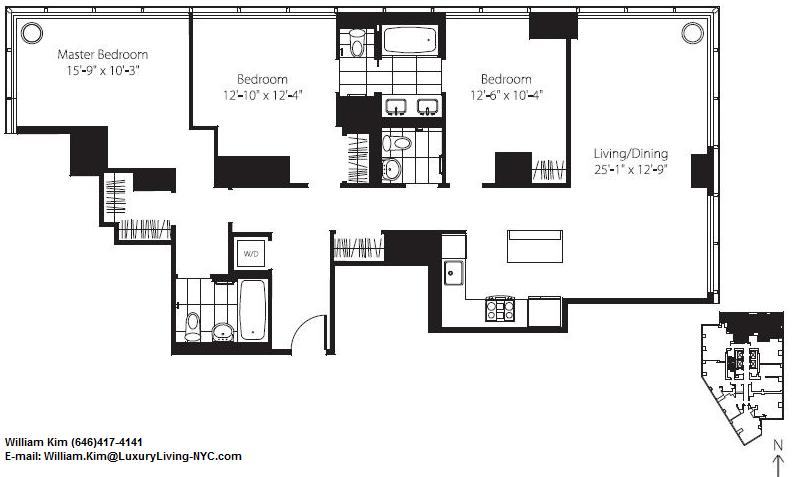Here is a detailed and cleaned-up caption for the image, describing the floor plan comprehensively:

---
Detailed floor plan of a house displaying:

- **Bottom Left Corner:** Contact information in black font - "William Kim 646-417-4141", with email "William.Kim@luxuryliving-nyc.com".

- **Top Left Corner:** Master bedroom measuring 15 feet 9 inches by 10 feet 3 inches. 

  Exiting the master bedroom, you enter the bathroom, featuring a toilet next to the door, a sink adjacent to it, and a full bathtub.

- **Right of the Hallway:**
  - Another bedroom measuring 12 feet 10 inches by 12 feet 4 inches directly to the right.
  - This bedroom has an en suite bathroom, with a toilet and divider separating the bathtub, and two sinks positioned opposite the bathtub.
  - This bathroom also connects to an adjoining bedroom, measuring 12 feet 6 inches by 10 feet 4 inches.

- **Proceeding from the Hallway:**
  - At the end of the hallway, you encounter the kitchen.
  - To the right of the kitchen is a spacious living room and dining room area.

This floor plan design is suitable for a seamless flow between private and communal living spaces, making it perfect for modern family living.
---